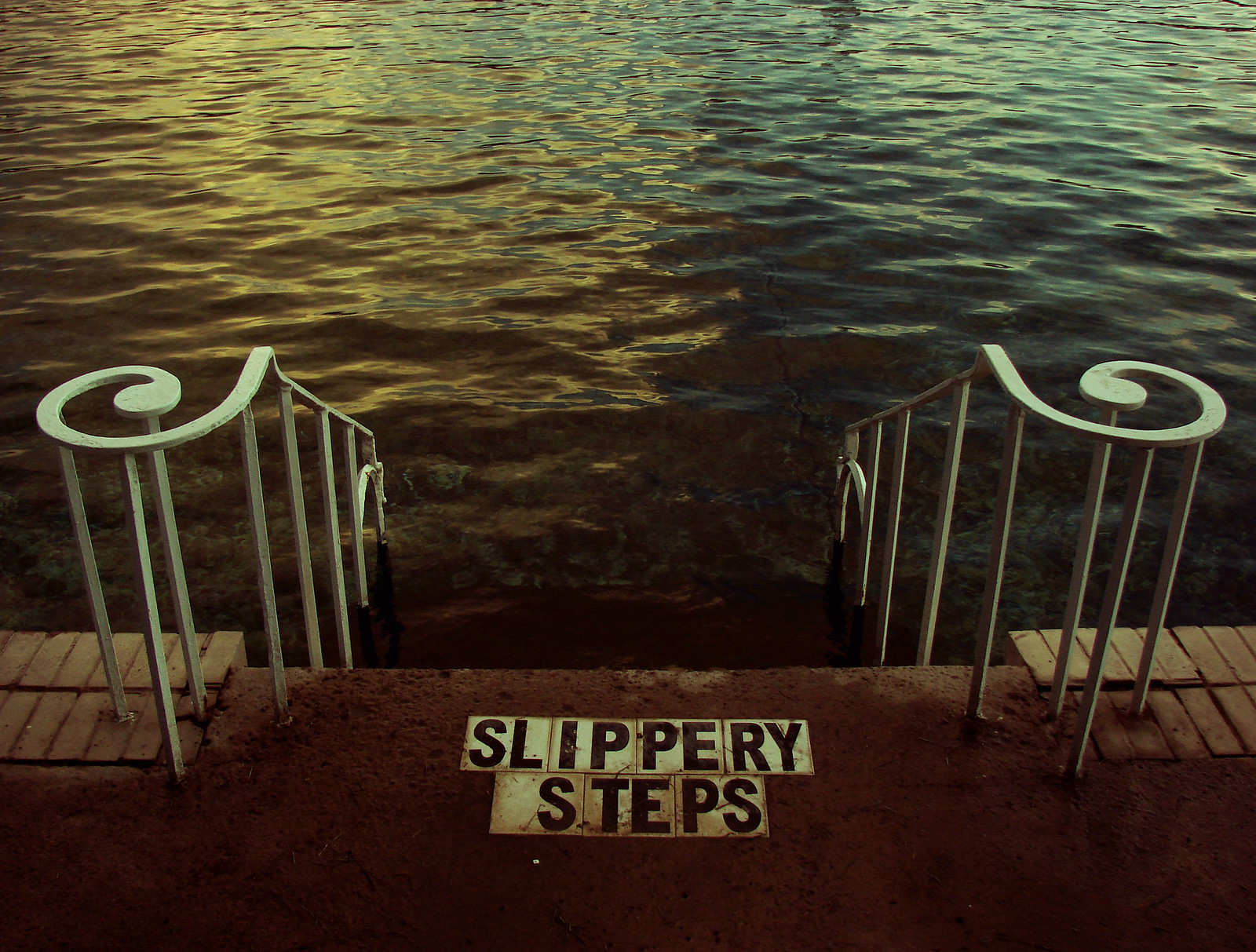The image is a color photograph in landscape orientation, depicting an old-fashioned staircase leading down into a murky body of water, possibly a lake or river. The staircase descends from a brick platform featuring a mix of red and gray bricks, with a damp and wet appearance. At the top of the steps, white tags with black, all-cap letters spell out "SLIPPERY STEPS," cautioning against the hazard posed by the wet steps. The staircase itself includes a central stone and brick structure flanked by iron railings on both sides. Each railing culminates in an elegant, decorative curlicue before plunging into the dark water, which ranges in color from black and gray to brown, with hints of blue. The lighting is very dark, accentuating the murkiness and sediment visible on the steps, and the overall atmosphere exudes a sense of antiquity and cautious forewarning.